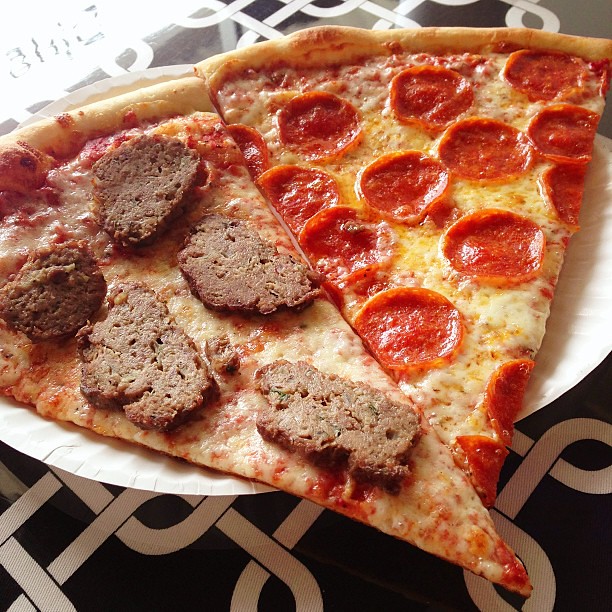The image features two thin-crust pizza slices on a white paper plate, positioned on a black cloth with a white fencing design. The slice on the right is a pepperoni pizza, generously topped with approximately 15 pieces of shiny, greasy pepperoni. The slice on the left is a cheese pizza adorned with five large slices of sausage, which appears to have some green seasoning inside. Both pizza slices are substantial in size, extending beyond the edges of the paper plate.